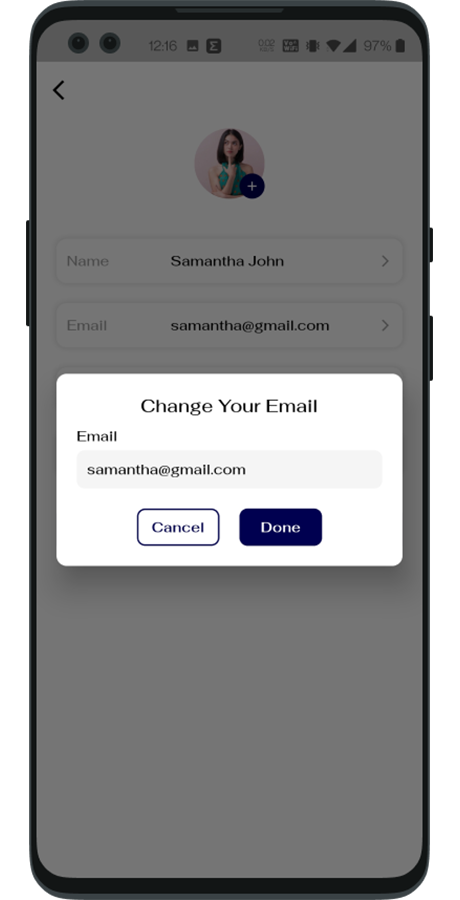The image displays a smartphone screen featuring an open contacts application. The focal point is a contact entry for a young woman named Samantha John. Her profile picture shows her with light skin, exhibiting a thoughtful yet playful expression as she rests her right index finger against her chin and gazes slightly off-camera.

The contact entry reveals Samantha's email as "samantha@gmail.com." An option to edit this information is prominently displayed, with a dialog box labeled "Change your email" allowing users to input a new email address or choose to cancel the action.

The interface has a clean design, predominantly with a white background. A back button is visible, although its destination within the app is unclear. Overlaid on this scene is a semi-transparent notification bar at the top of the phone screen. It indicates the device is on vibrate mode, has full signal bars and Wi-Fi connectivity, and a battery level of 97%. Multiple app notifications are present, though their specific details are not discernible.